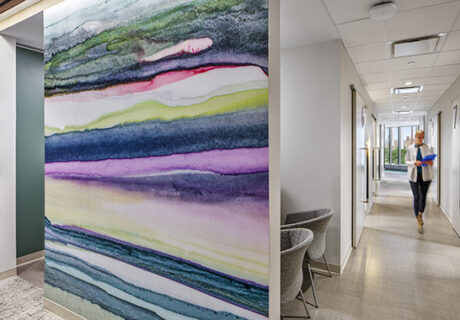The image depicts a modern office interior, likely a photograph rather than a digital rendering. The scene features a prominent, tall wall on the left, painted in a striking watercolor style with sweeping horizontal bands of pale blue, green, dark blue, white, purple, yellow, and other hues, giving it a mural-like appearance. This wall partially encloses a small office area equipped with two comfortable, gray fabric chairs with taupe-colored metal legs. 

To the right of the mural wall extends a long, beige laminate-floored hallway, with neutral white and creamy walls, and a white drop ceiling adorned with square lights. Walking down this corridor towards the front of the image is a woman with blonde hair, dressed in a white jacket and dark pants, holding a blue clipboard. The hallway is lined with doors on both sides and has a view of windows at its far end, suggesting that it leads to an exterior area. The overall setting, with its modern furnishings and neutral color palette, resembles a professional office environment, potentially a doctor's office.